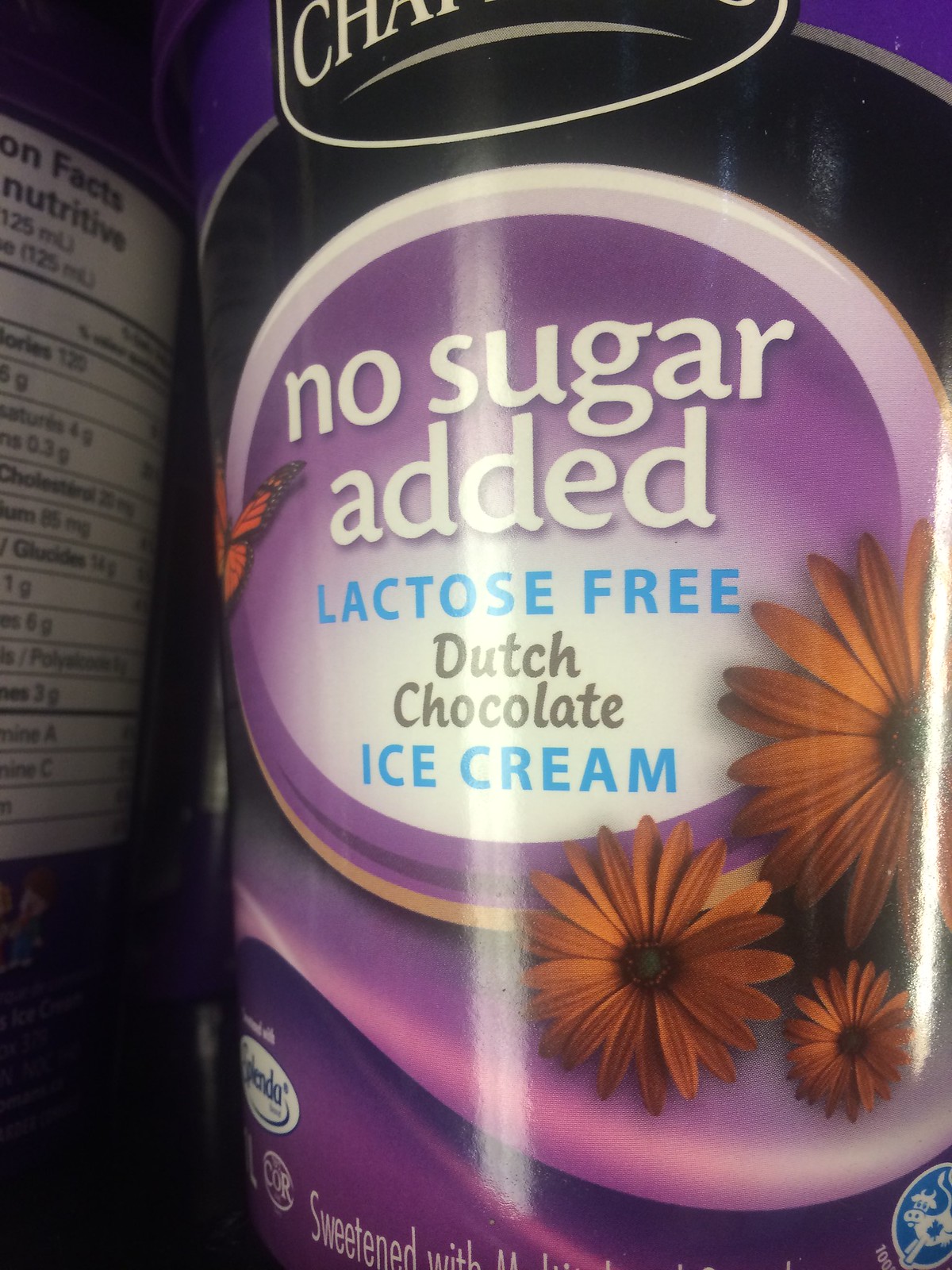In this rectangular close-up photograph, the focal point is a container of ice cream with a distinctively designed label. The top portion of the container is a dark blue hue, transitioning to a vibrant purple below. Centrally located on the container is a label, encircled in white with a purple background, which clearly states, "No sugar added, lactose-free, Dutch chocolate ice cream." Adjacent to this main label, in the lower right-hand corner, sit three delicate daisies. On the lower left side within an oval white background, the word "Splenda" is prominently displayed. Moreover, towards the bottom of this ice cream container, the phrase "sweetened with" is visible, leading the eye to the lower right corner where there is an image of a white cow inside a blue shape with a white border.